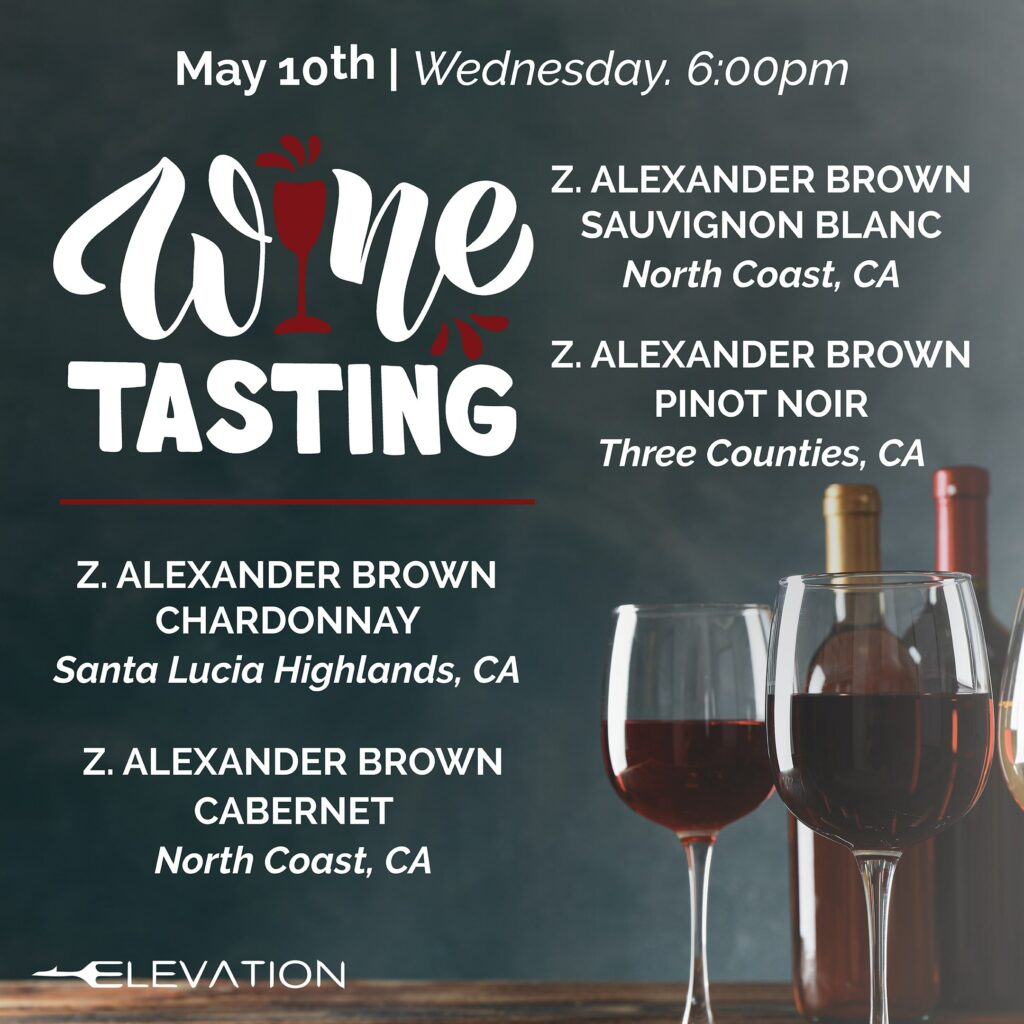This image is an advertisement for a wine tasting event scheduled for May 10th, Wednesday at 6 p.m. The background features a bluish hue, and at the top of the ad, the date and time are displayed in white text, while "Wine Tasting" is written in big, curly letters with the "I" cleverly replaced by a red wine glass. The advertisement highlights a selection of wines from Z. Alexander Brown, including Sauvignon Blanc from North Coast California, Pinot Noir from Three Counties, California, Chardonnay from Santa Lucia Highland, California, and Cabernet from North Coast, California. In the bottom left-hand corner, the word "Elevation" is displayed, with the first "E" ingeniously designed in the shape of a fork with three prongs. On the right side of the ad, there are two wine glasses filled halfway with red wine and two wine bottles behind them, one capped in yellow and the other in red.